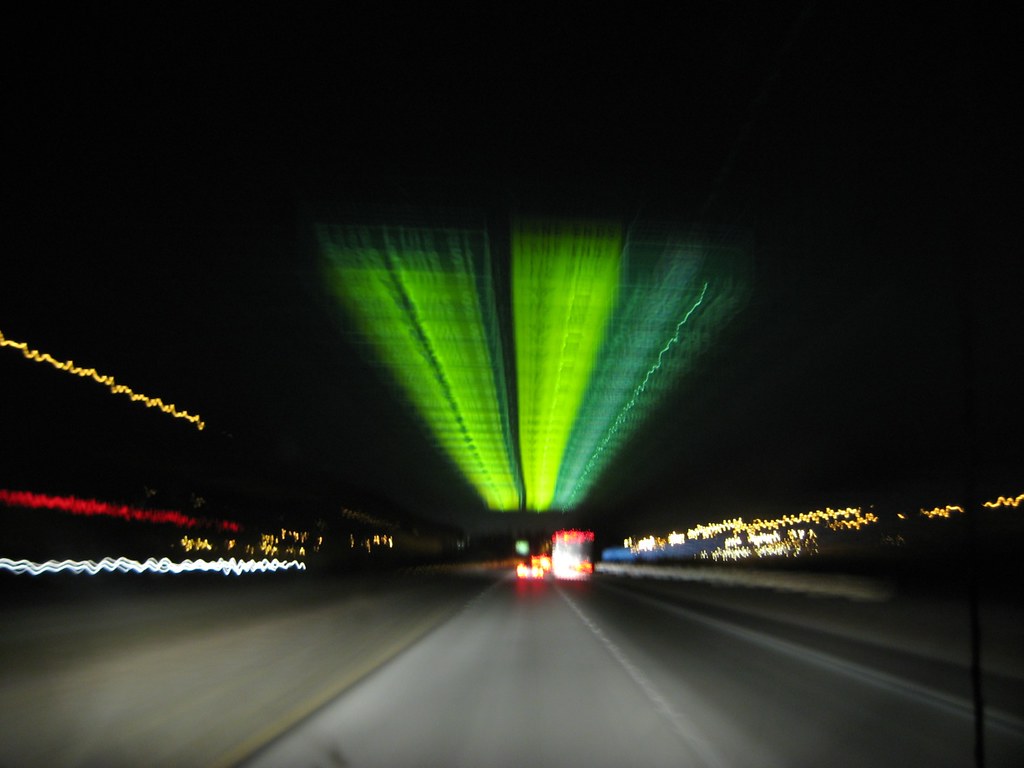A nighttime scene captures a gray road illuminated by the headlights of approaching vehicles. On the right-hand lane, a bus is prominently visible, while cars occupy the left lane, their red taillights glowing vividly. One vehicle, ahead of another in the left lane, displays distinct markings: two lime green stripes flanked by a darker green stripe running along its side. The road appears uniformly flat, and the far lanes remain indistinct. Streetlights line both sides of the road, casting a mixture of light. On the left side, a dynamic streak of red and yellow light cuts through the scene, contrasting with clearer, white lights on the right, accented by a soft blue glow in front of them.